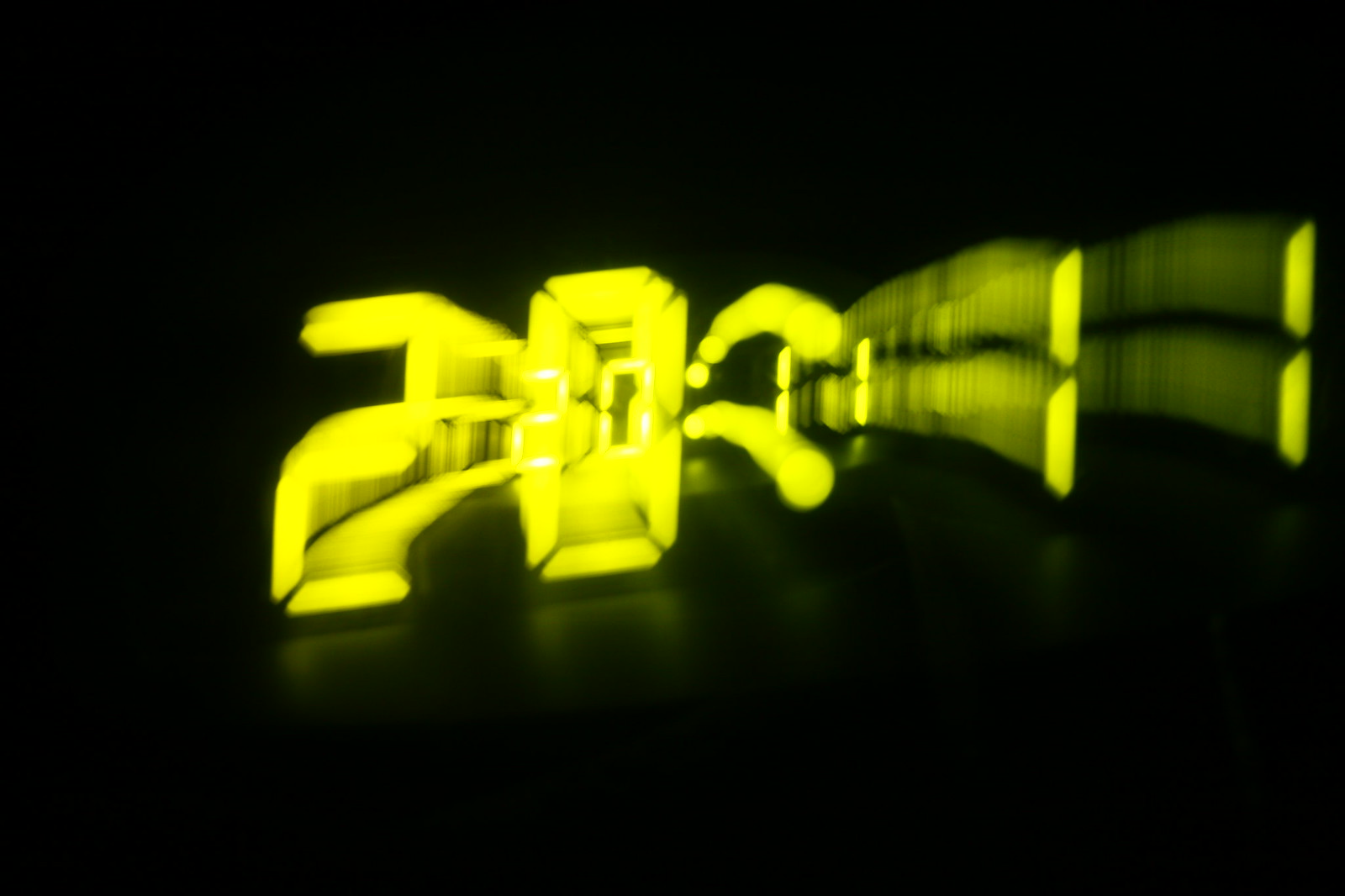A striking nighttime photograph captures the ethereal beauty of light in motion. The image showcases the digital numbers "20.11" illuminated in a vibrant yellow against a stark black background. Due to a long exposure and slow shutter speed, these numbers appear blurred, trailing through space and creating a dynamic, almost ghostly effect. The interplay of darkness and luminescent digits forms a mesmerizing composition, highlighting the transient nature of light and movement in a single, captivating frame.